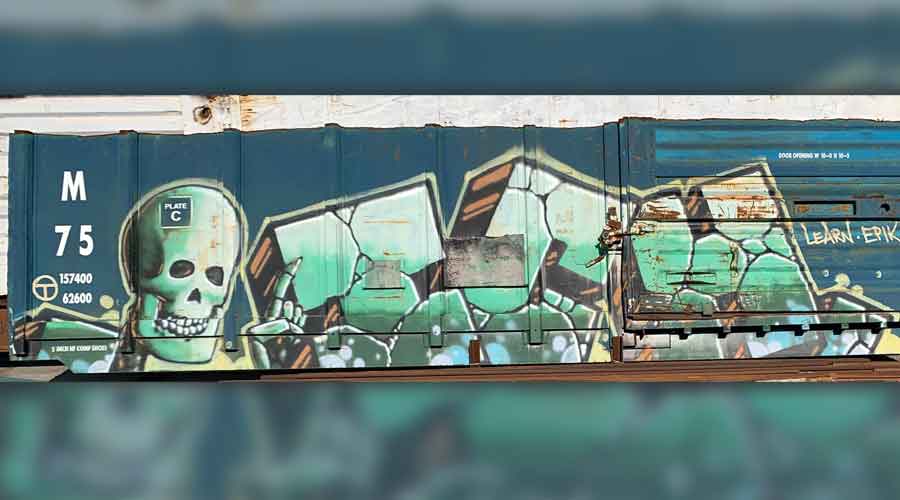The photograph captures a vivid piece of graffiti on the side of a bluish shipping container, possibly train cars. The graffiti features a detailed, green and white skull on the left side, which includes a skeleton with its index finger pointing upwards while the rest of the fingers are together. To the right of the skull, there are block-like letters in green and white, accented with orange and black. Above the graffiti, the text "M75" is clearly visible, with additional identification numbers "157-400-62600" below it. The artwork also includes the label "plate C" near the skull. The background above the container suggests a clear blue sky.